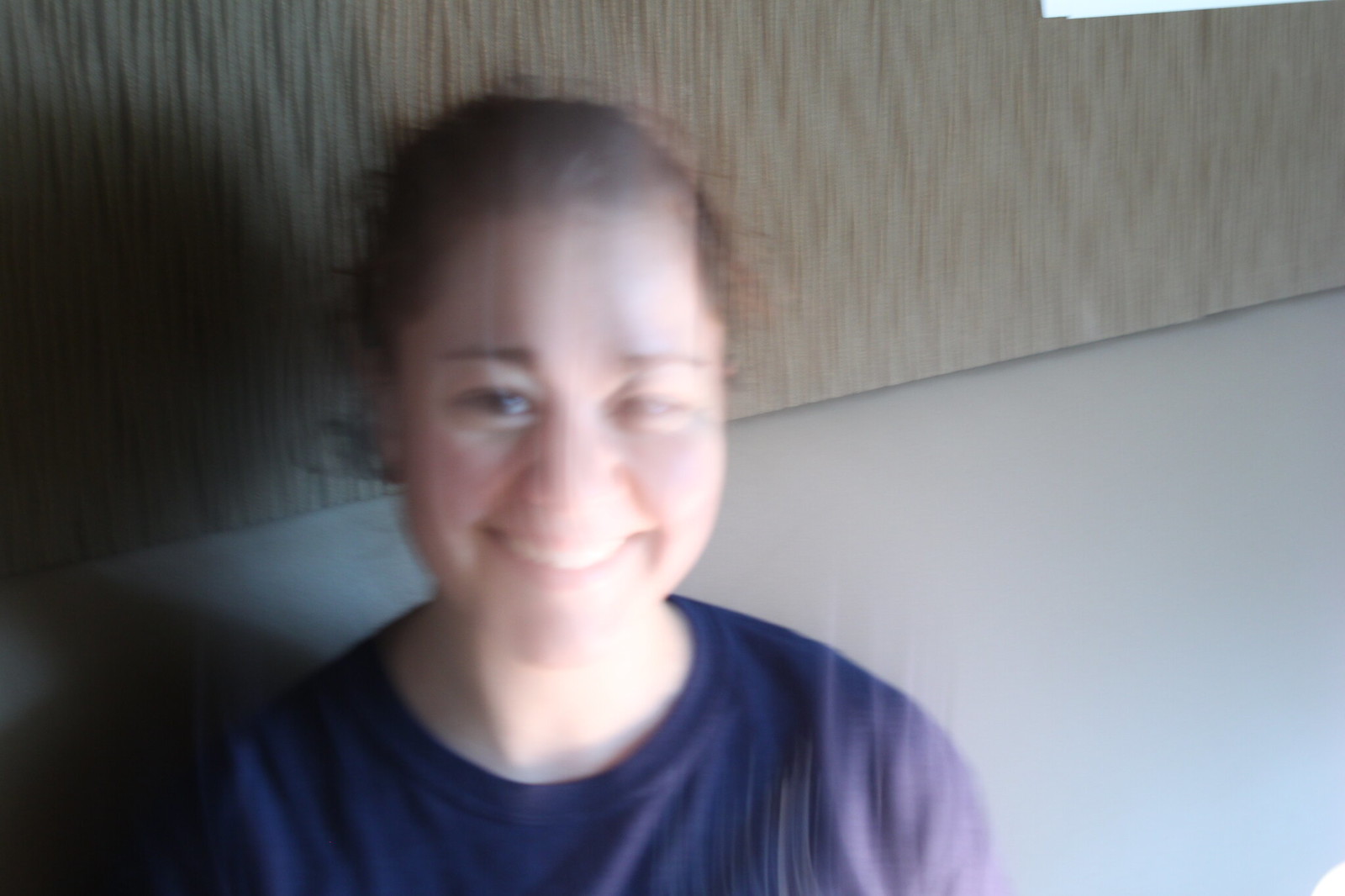The photograph captures a slightly blurry image of a smiling woman with brown hair and presumed brown eyes, seated in what appears to be a booth. The rectangular frame of the image extends horizontally. The woman, with fair skin, gazes directly at the camera, radiating cheerfulness. Her arms are not visible as they rest by her sides. She is dressed in a blue shirt, which contrasts with the white material of the booth she is sitting in. The background above the booth features a brown material, possibly wallpaper. Light enters the scene from the right, casting distinct shadows. This illumination creates a stark light-and-shadow effect, leaving the left side of the woman's face in a shadow while brightly lighting the right side. A deep shadow forms behind and to the left of her, highlighting the direction of the light source.